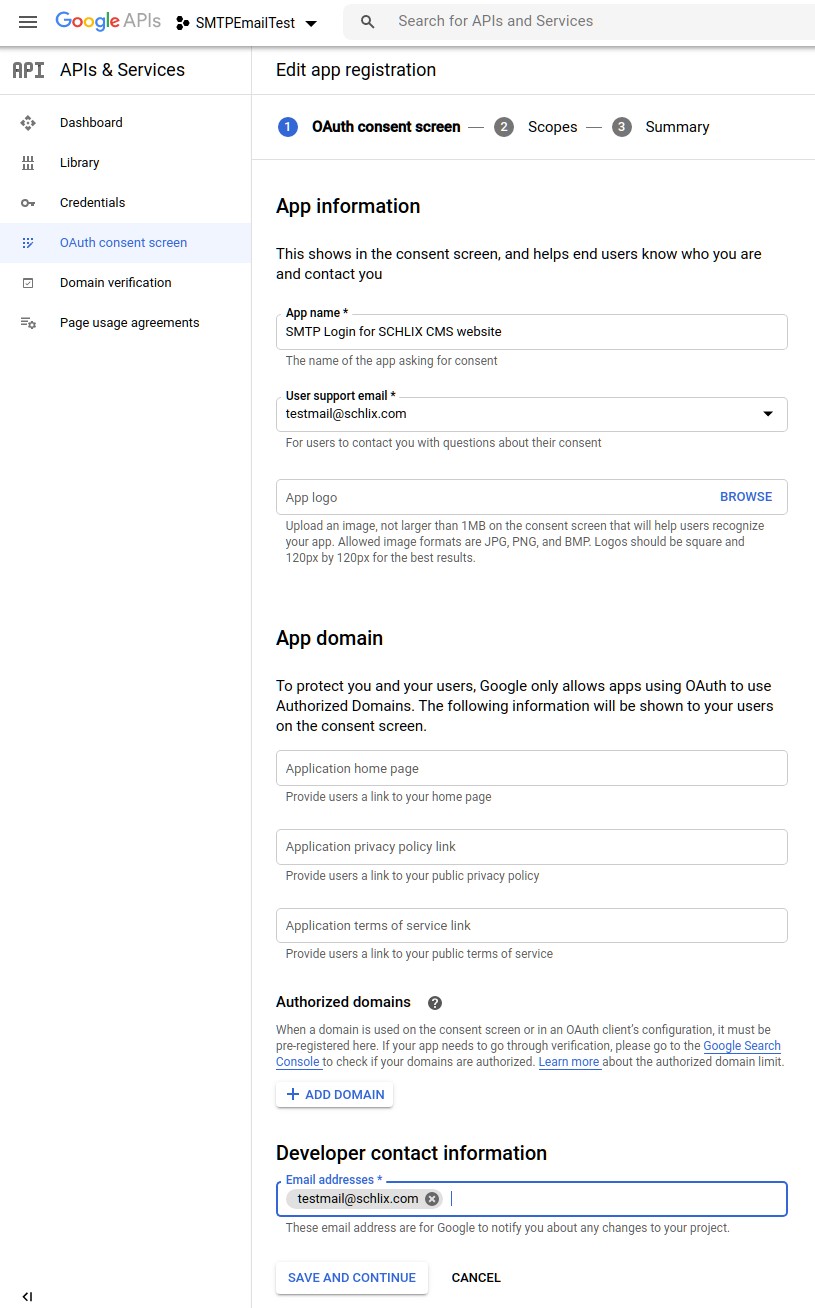The image depicts an interface from the Google APIs website. At the top right corner, there is a menu labeled "Google APIs." A section labeled "SMI something test" is partially visible. Below the top menu bar, a search bar is present. Directly underneath, the interface is divided into sections labeled "API," followed by "APIs & Services." Key menu options are listed including "Dashboard," "Library," "Credentials," "Auth," "Domain Verification," and "Page Usage Agreement." On the right side of the interface, there is an "Edit App Registration" option, which includes subsections "Auth Consent Screen," "Scopes," and "Summary." Further down, there are fields for "App Information" and "App Domain," accompanied by various dropdown menus. Below these fields is a section for adding "Authorized Domains," with an option to input and add a new domain. At the bottom, there is a "Developer Contact Information" section. Two action buttons, "Save and Continue" and "Cancel," are available for form submission or cancellation.